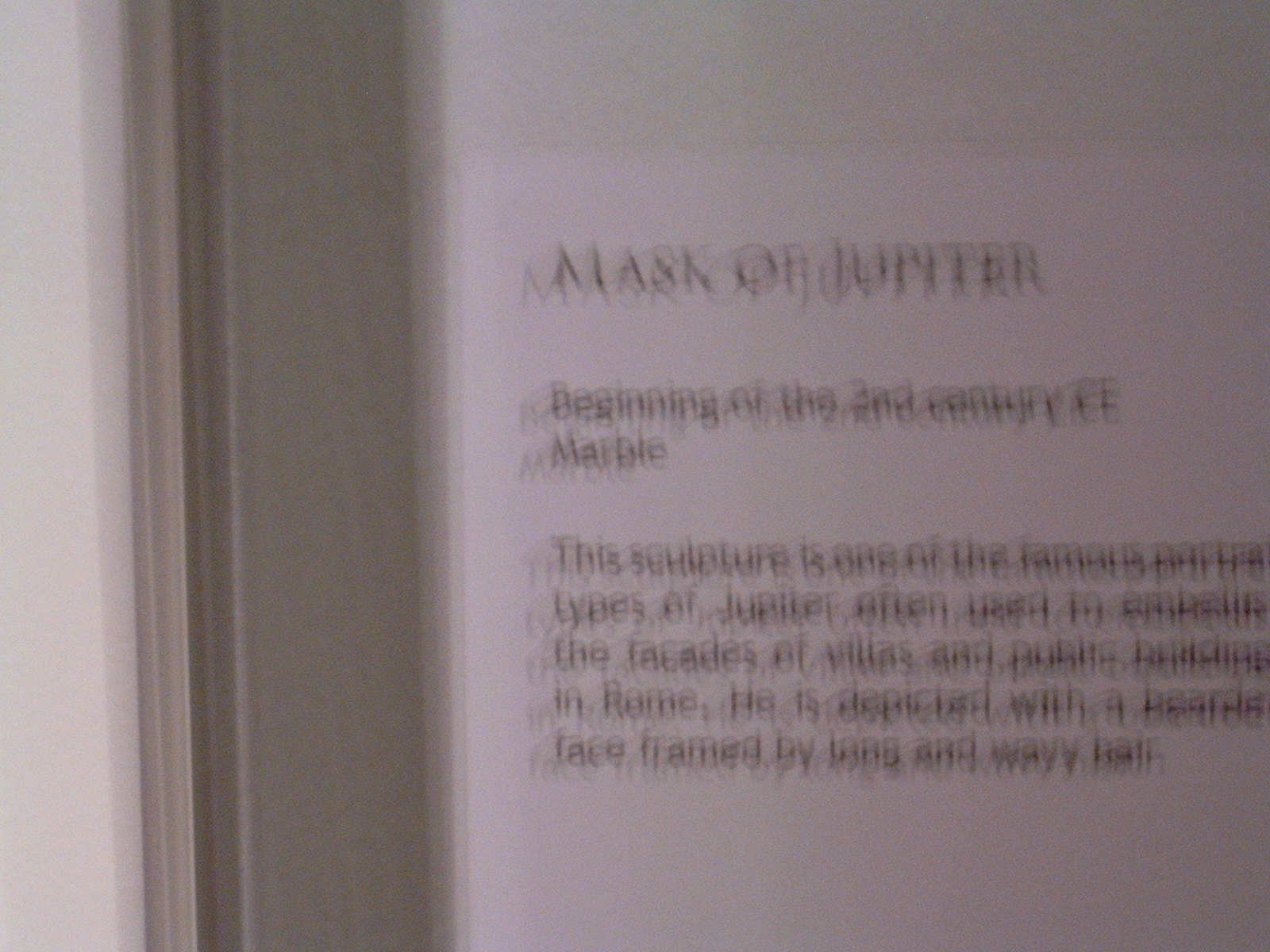Here is the cleaned-up and detailed caption for the image:

---

This highly blurred image captures a marble sculpture from the 2nd century CE, identified as the "Mask of Jupiter." Despite the blur, the accompanying inscription can be read. It describes the sculpture as a notable portrayal of Jupiter, the Roman god, often adorning the facades of villas and public edifices in Rome. The sculpture features Jupiter with a bearded face and long, wavy hair. Although the mask itself is not visible due to the image's poor quality, the detailed description on the inscription provides a vivid depiction of this classical artwork.

---